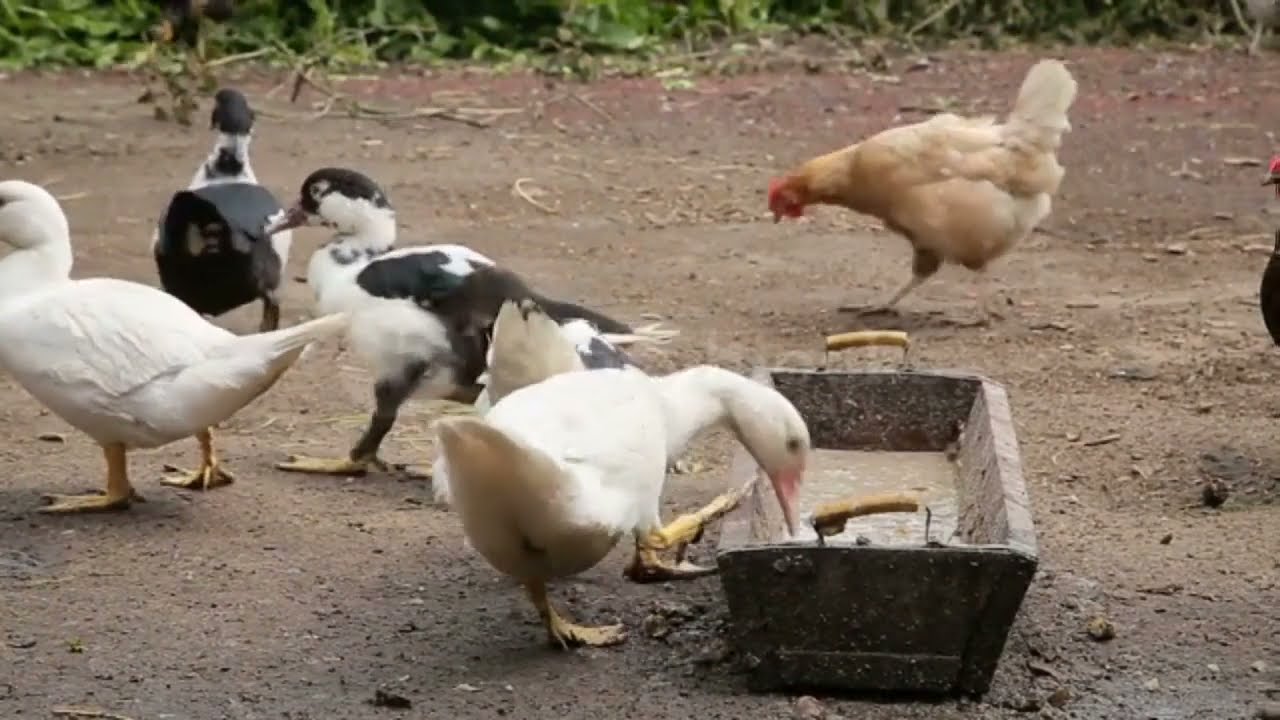The photograph captures an overcast day on a farm with several fowl milling about on a muddy dirt ground. Central to the image is a short, metallic trough with wooden handles wrapped in white, containing a mixture of sludge and mud. A white duck with yellow feet is feeding from the trough, facing to the right. To the left, a black and white splotchy duck is walking away, while another white duck is seen moving in the same direction. The backside of an additional black and white splotchy duck is also visible as it heads towards the far edge of the scene, where a patch of greenery is just visible. Directly behind the trough, a chicken with a red comb and predominantly white feathers, along with a brown belly, walks across the ground. Overall, the scene features a diverse mixture of domesticated birds casually engaging with their surroundings.